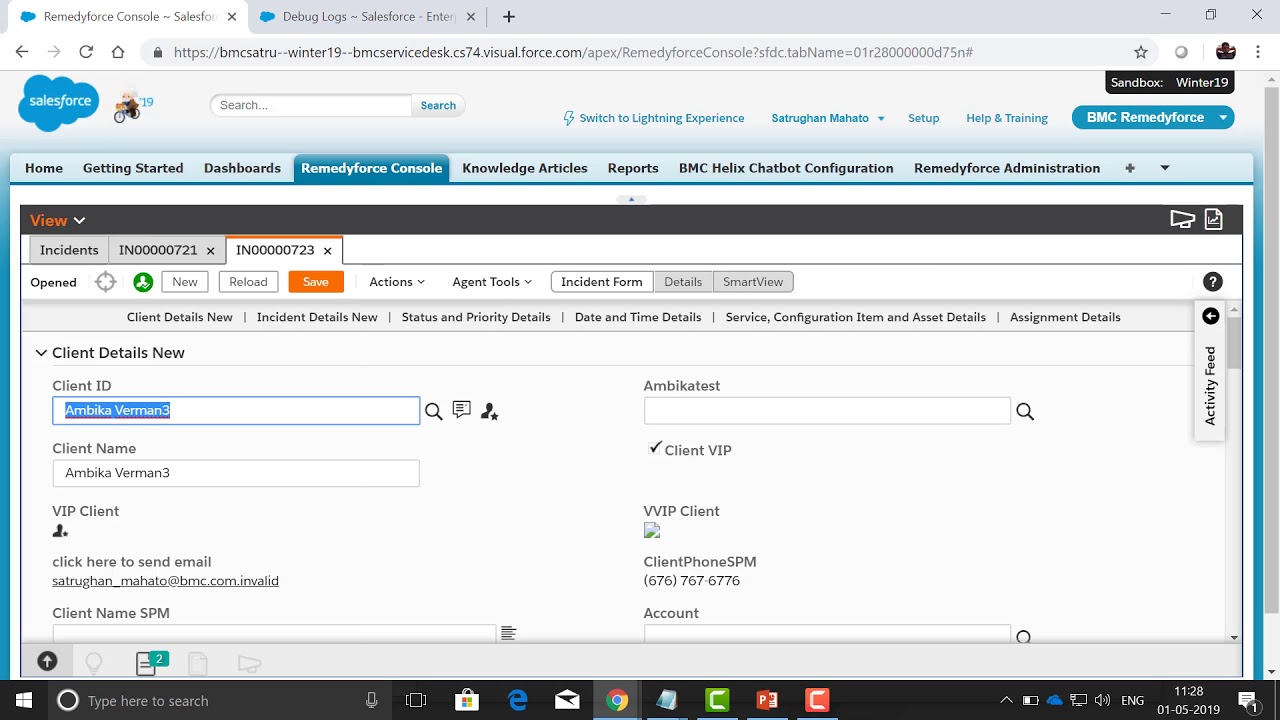Screenshot of a Website: Comprehensive View of the Regain Force Console Interface

Captured in this image is a detailed screenshot of a computer screen displaying the "Regain Force Console" website. 

**Top Section:**
- **Upper Left-Hand Corner:** The title "Regain Force Console" is prominently displayed. Adjacent to it is another tab labeled "Debug Loss Salesforce," which is not highlighted, indicating it is inactive.
- **Address Bar:** The Internet address bar below displays the URL "bmcsatru-119."
- **Text Box and Icons:** Below the address bar, there is a text box featuring the Salesforce icon on the left and an icon of a person riding a bike, next to a search box. This section also contains links and options for "Switch to Lightning Experience," "Setup," "Help and Training," and "BMC Regain Force" which is displayed in a blue elongated oval with white text.

**Primary Navigation:**
- **Headers and Tabs:** A navigation bar outlines various headers: "Home," "Getting Started," "Dashboards," "ReadyForce Console," (which is highlighted), "Knowledge Articles," "Reports," "BMC Hedge Chat Point Configuration," and "Regain Force Administration." 

**Main Content Section:**
- **Form:** A partially filled-out form labeled "View" is visible. 
- **Instances:** Tabs below the form include "Instance" and specific instance IDs such as "IN0000721" and "IN00000723" with the latter being highlighted.
- **Labels:** The form contains several action buttons and labels like "New," "Reload," "Save," "Actions," "Agent," "Tools," "Instant Form," "Details," and "Smart View."

**Client and Incident Details:**
- **Detailed Views:** Further sections labeled "Client Detail Views," "Incident Detail Views," "Status and Priority Details," "Game Time," "Service Configuration Items," "Asset Details," and "Assignment Details" appear below.
- **Client Information:** Section for "Client Detail Views" includes input fields for "Client ID," "Client Name," "Client Phone Number," and "Client Email."

**Lower Section:**
- **Icons and Taskbar:** The bottom section of the screen displays multiple icons such as "Internet Explorer," "Google," and several others. The taskbar reveals the "Start Menu" at the bottom left-hand corner and system notifications like "Battery," "Cloud Connection," "Language," and "Date and Time" at the bottom right-hand corner. 

This image provides a comprehensive overview of the Regain Force Console interface, showing navigational elements, active sections, and pertinent details for managing and viewing instances and client information.